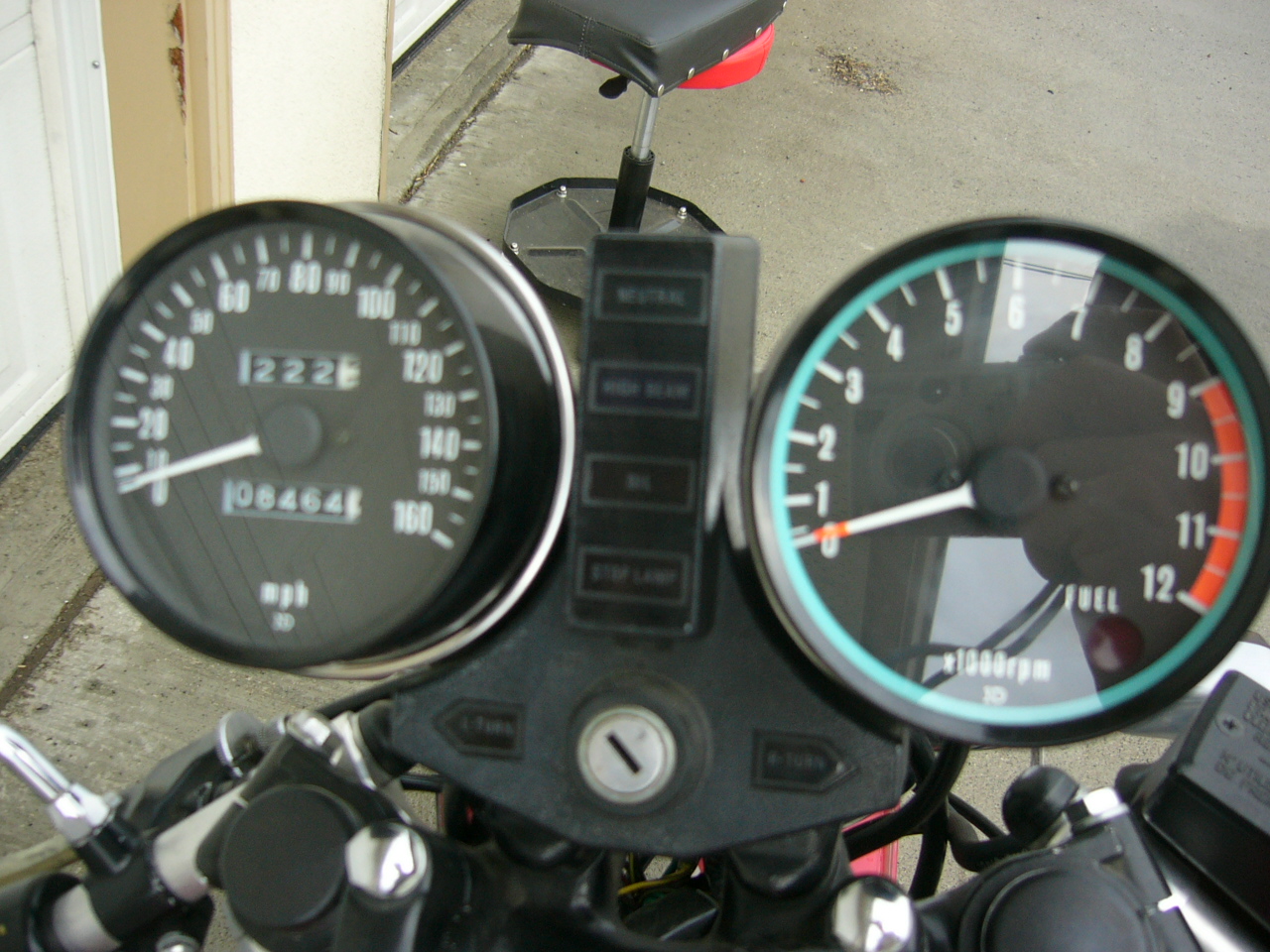The image showcases the intricate front view of a motorcycle against a mixed backdrop, featuring elements of urban and rustic settings. The right side of the frame reveals a gray cement surface, while the left side is flanked by gray wooden planks. In the upper left corner, a white and tan building with hints of red peeks into the shot, adding a splash of color to the composition.

Central to the image is the motorcycle’s control panel. At the top, a black structure with a red underside catches the eye. Connected by a metal bar, the motorcycle seat features a black adjustment mechanism. Below, an area with black circular shapes stands out, hinting at key components of the motorcycle.

The handlebars and dashboard command attention with two prominent circular gauges. The left gauge, encased in black and gray with silver accents, is peppered with numbers and dashes. The thicker dashes at the numbers contrast with the thinner ones in between. Above, a counter displays "222" in light green on a black background, accompanied by another counter showing "06464" in light blue and black, supplemented by the label "MPH."

On the right, the second gauge mirrors the left, outlined in black and green. Numbers dominate the face, with longer, bolder dashes at the numbers and finer dashes in-between. A red curved line marks the space between the 9 and 12 positions. Topping the gauges, a black rectangle houses variously colored indicators—green, blue, red, and a deep purple—each labeled with unreadable text due to their size.

The entire control panel is framed by a black shape, spreading outwardly to encompass the gauges, creating a cohesive design. Notably, there is a key slot and directional arrows on either side—left on the left and right on the right—along with a visible handbrake, hinting at the intricate functionality of the motorcycle.